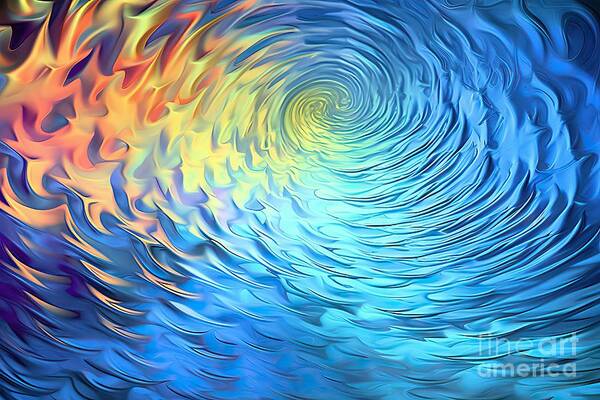The image is a detailed digital painting resembling an optical illusion, prominently featuring a vortex of swirling colors. At the center of the spiral, there is a deep blue, reminiscent of water funneling into a whirlpool. This blue extends predominantly to the right side of the image. As the swirling motion progresses outward, it transitions into vibrant hues of yellow, orange, and various shades of reddish-orange flames. Towards the left side, these colors turn into a yellow-green tint, blending harmoniously with the central blue. The quality of the image is high, and the entire composition creates a mesmerizing, almost illusionary effect. On the bottom right corner of the painting, the words "The Art America, Fine Art America" are clearly visible in white text. No other details such as the artist's name or additional text are present in the image.